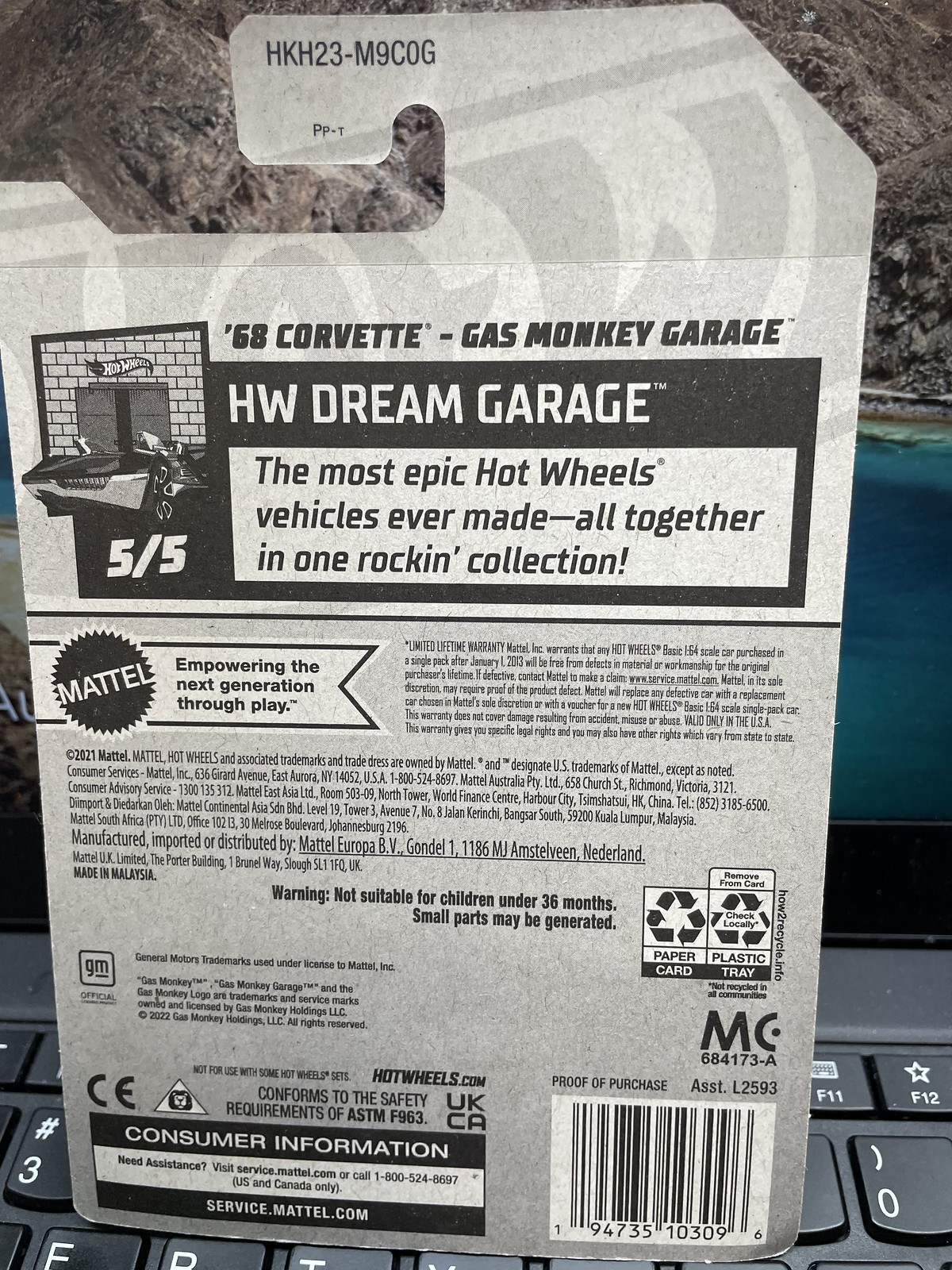The image depicts the backside of a rectangular cardboard packaging for a Hot Wheels product, placed on top of a laptop keyboard. The prominent text on the packaging reads "68 Corvette Gas Monkey Garage" and "HW Dream Garage: The most epic Hot Wheels vehicles ever made all together in one rocking collection." The packaging is predominantly gray with black and white text, and features a hook at the top for hanging display.

Further details on the back include extensive product information: a large headline area with the Hot Wheels logo at the top left corner, rating of 5 out of 5, consumer information, and a warranty notice. The packaging specifies a code at the top "HKH323-M9COG," and below it, a description of the product alongside logos such as Mattel and various recycling symbols. There is a section labeled "Empowering the next generation through play," and a warning about the suitability for children under 36 months due to small parts. 

Additional details include contact information for Mattel's consumer services across various regions, such as the USA, Australia, East Asia, India, South Africa, and Europe. The packaging also has hazard symbols and recycling instructions, alongside trademarks and legal information regarding the owners of Gas Monkey Garage and General Motors.

The bottom right corner of the packaging features a barcode and proof of purchase code "S ST.L25 M3," as well as compliance logos indicating conformity to ASTM F963 standards and UKCA. The entire scene, with the packaging sitting on the laptop keyboard, showcases visible laptop keys and part of the screen in the background.